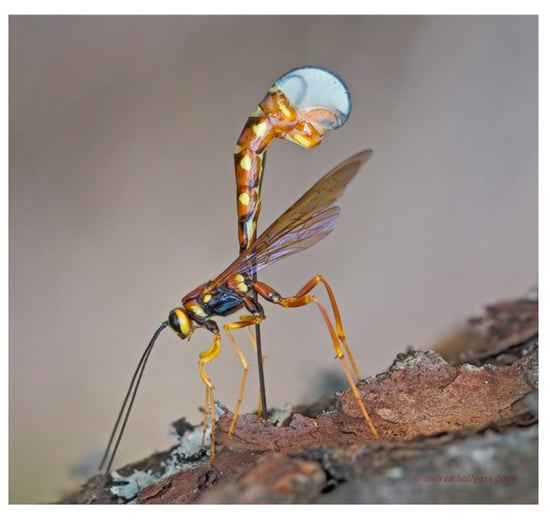This very close-up photograph captures a striking insect in vivid detail. The insect, which appears to have characteristics of a wasp, boasts a yellow and black body with two prominent, long, black antennae extending from its head. It stands on what seems to be tree bark, displaying its stilt-like legs that are a blend of orangish yellow and gold. Its body is adorned with black, yellow, and brown stripes, giving it a distinctive appearance. The insect is poised with its body hunched over, supported by four long legs, and its head marked by a contrasting yellow bottom and black top.

Emerging from its back are two large, nearly transparent brown wings, detailed with visible veins. From the end of its body, a thin, sharp rod extends, terminating in a bulbous, clear structure that resembles a water droplet. This structure is attached to a segment of the body that combines brown, orange, and yellow hues, tapering into a slender black base.

The insect is set against a blurred background of beige earth tones, contributing to the overall focus on the detailed foreground. The surface it rests on appears to be a mixture of gray, red, and orange, resembling roof tiles or bark sprinkled with snow. Additionally, a subtle watermark in red is visible at the bottom right corner of the image, completing the composition.